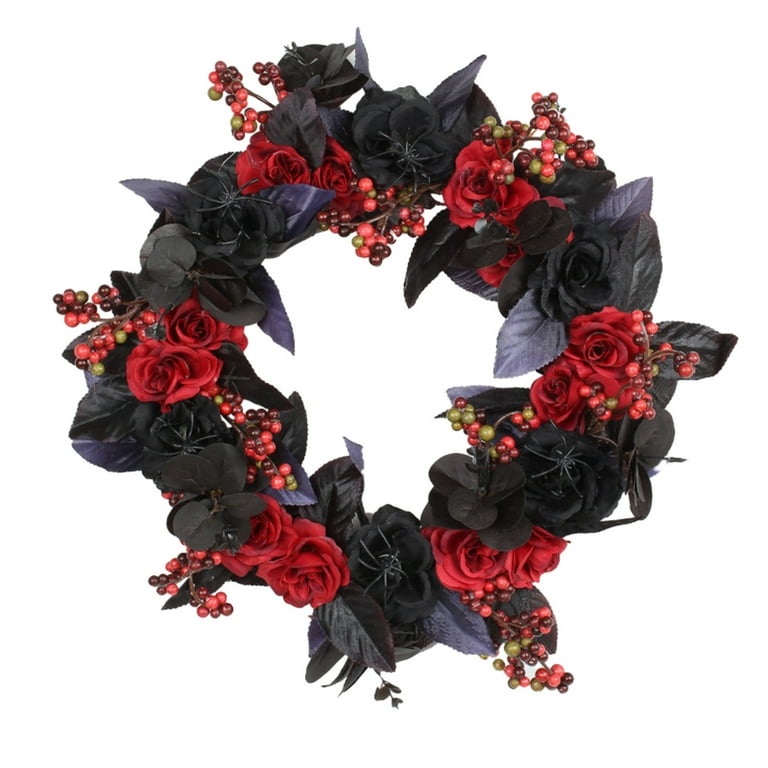This image features a medium-sized, circular wreath set against a solid white background. The wreath is crafted in a striking, gothic style, designed for year-round display, possibly suitable for a front door. The wreath boasts six clusters of roses, each consisting of two paired roses. The rose pairs alternate between vibrant red and deep black hues, creating a stunning contrast. Interspersed among the roses are clusters of holly berries in a palette of green, pale red, and dark burgundy, adding a rich, textured accent. Gray and black leaves weave throughout the arrangement, enhancing its dark, elegant aesthetic. Adding to the wreath's unique character, plastic black spiders are perched on some of the black roses, contributing to a slightly eerie yet stylish flair.